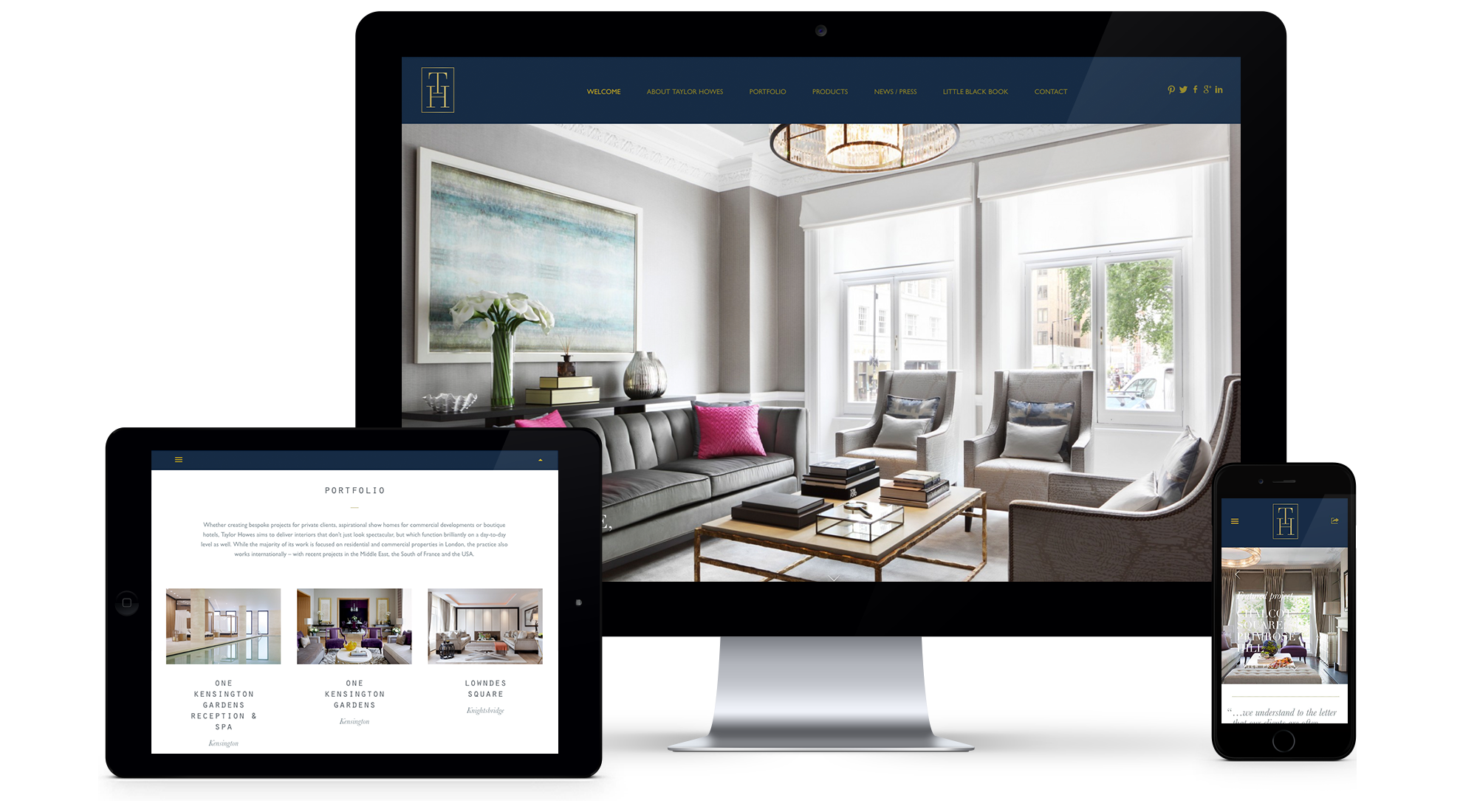This image showcases a sophisticated home design application, prominently displayed on three different devices: a large PC screen, a tablet on the left, and a smartphone on the right. The app’s branding features the initials "TH," elegantly designed with an inner triangle intersecting a "T" at the top and an "H" at the bottom. 

The central focus of the app display is a stunning lounge area, furnished with stylish grey couches adorned with exquisite pillows and complemented by elegant overhead lighting. The interface suggests that the application is intended for interior design, offering users a detailed view of well-designed living spaces.

The top navigation bar includes various options: "Welcome," "About," "Take Homes," "Portal," "More Products," "News," "Utility," "Black Book," and "Contact." Additionally, social media icons for Pinterest, Twitter, Facebook, Google, and LinkedIn are present, emphasizing the app’s connectivity and social sharing capabilities.

Each device screen displays different room designs within the app; while the primary PC screen features the beautiful lounge, the tablet and smartphone screens showcase alternative spaces, with what looks like a pool room featured on one of the devices. This exemplifies the app’s versatility in displaying various home design concepts across multiple platforms.